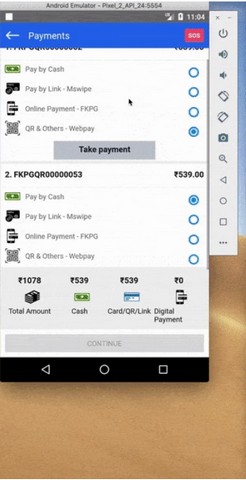In this screenshot, captured from an Android Emulator running on a Pixel 2 with API level 24, you can observe several on-screen elements in detail. At the very top center, there are light gray words reading "Android Emulator Dash Pixel 2 Underscore API Underscore 24 5554." Moving to the upper right corner of the emulator screen, the current time of the screenshot is displayed as "11:04," with a white battery icon to its left showing the battery status, and a 2-bar phone signal strength icon further to the left.

Directly below this row, in a small, neatly boxed area, the word "Payments" appears on the left side accompanied by a left-pointing white arrow. On the far right of this boxed area is the label "SOS." 

Under the "Payments" section, there are multiple categories listed in sequence. The categories are:
1. "Pay by Cash"
2. "Pay by Link"
3. "MSWipe"
4. "Online Payment"
5. "FXPG"
6. "QR and Others"

Each category has a corresponding blue circle to its right. Notably, only the circle next to "QR and Others" is filled in, while the circles for the other categories remain unfilled.

At the bottom of the listed categories, inside a small box with a grey background, the phrase "Take Payment" is written in black text.